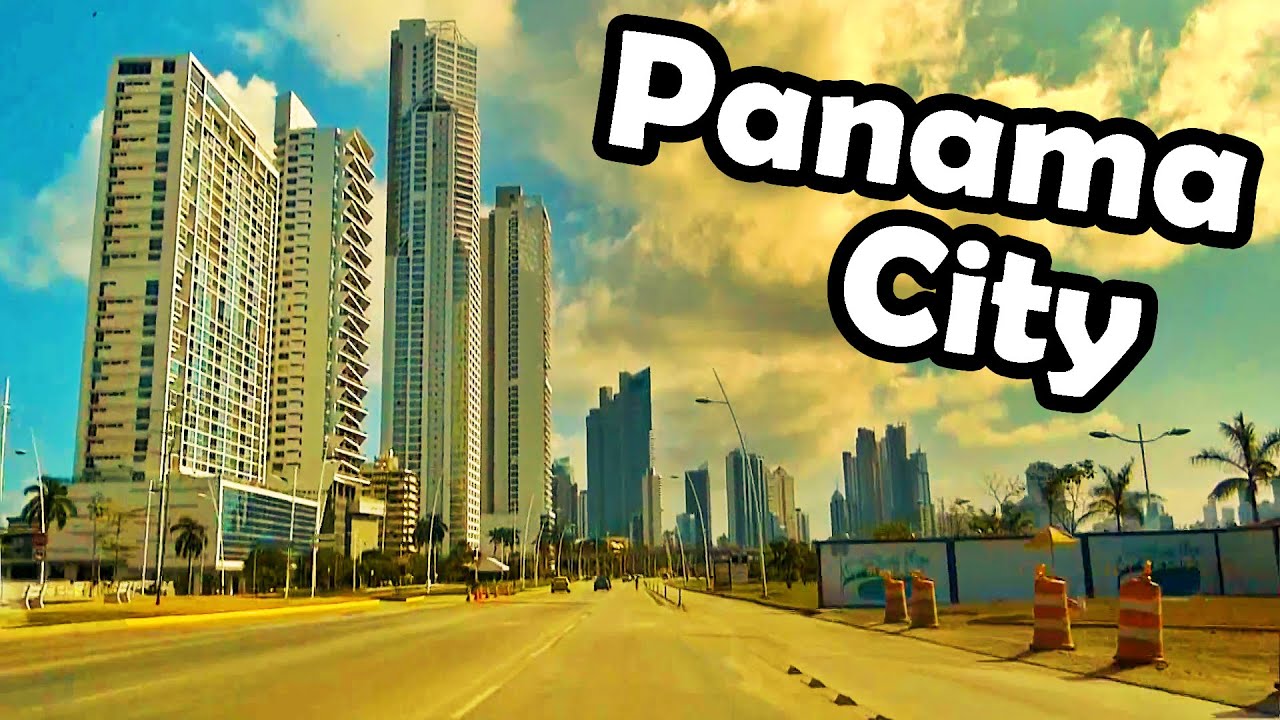In this hyper-realistic video game screenshot, reminiscent of the Grand Theft Auto series, the vibrant cityscape of Panama City is showcased. Dominating the right-hand side of the image is the text "Panama City," rendered in bold white letters with a black outline. The scene is bathed in natural light, with a bright blue sky dotted with fluffy white clouds overhead. Numerous palm trees line both the left and right sides of the image, adding a tropical touch to the urban environment.

To the left and stretching into the background, a cluster of towering skyscrapers define the skyline, hinting at the city's bustling activity. In the foreground on the right, orange construction barrels suggest ongoing development or roadwork. Several cars navigate a two-lane street that cuts through the scene, highlighting the infrastructure and daily flow of traffic. Murals decorate the sides of buildings, particularly one on the right-hand side and another on the facade of a prominent skyscraper, adding a layer of cultural texture and artistic expression to the cityscape.